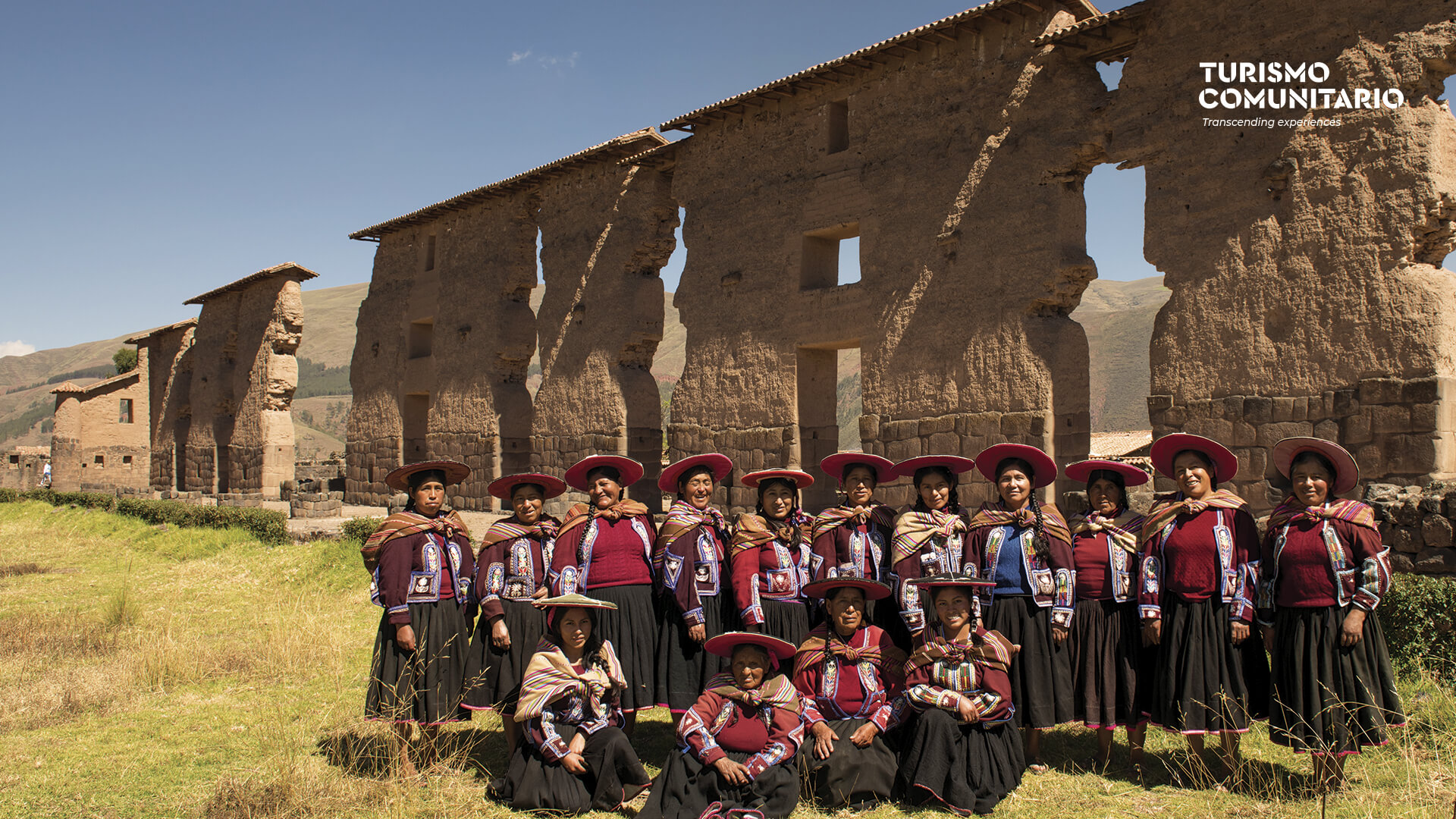In the foreground of this countryside setting, a group of native women, dressed in coordinated traditional attire, pose for a photo. They are lined up with four seated in front and the rest standing shoulder to shoulder behind them. Each woman wears a long black skirt with red trim, a burgundy knitted sweater adorned with designs along the lapel and wrists, a scarf draped around their shoulders, and a wide-brimmed sombrero-like hat in a reddish hue. The women stand on a grassy field. Behind them, extending diagonally from the top right corner to the left, are the large, fragmented remains of an ancient structure made of light brown stone. The walls feature gaps where doorways and windows once stood, hinting that the building was once three stories high. The sky above is a mix of forest green, blue, and sky blue hues. In the upper right corner of the image, the text “Turismo Comunitario: transcending experiences” is displayed in white.